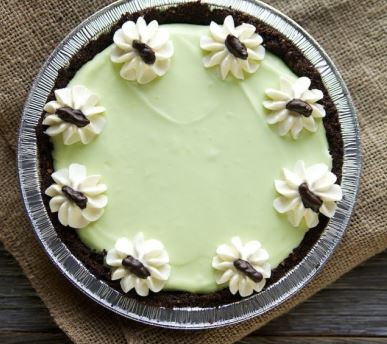The image displays a dessert in a round aluminum pie pan, seated on a light brown fabric, which in turn is placed on a dark wooden table. This dessert, possibly a pie or cake, is adorned with intricate decorations. The center features a wide expanse of green icing, surrounded by a contrasting dark chocolate-colored edge. Encircling the dessert are eight flower-like designs made from white icing, each with a bean-shaped, chocolate-like stamen in the middle. The overall presentation is both visually appealing and precise, highlighting the artistic arrangement of the floral motifs against the simple backdrop.